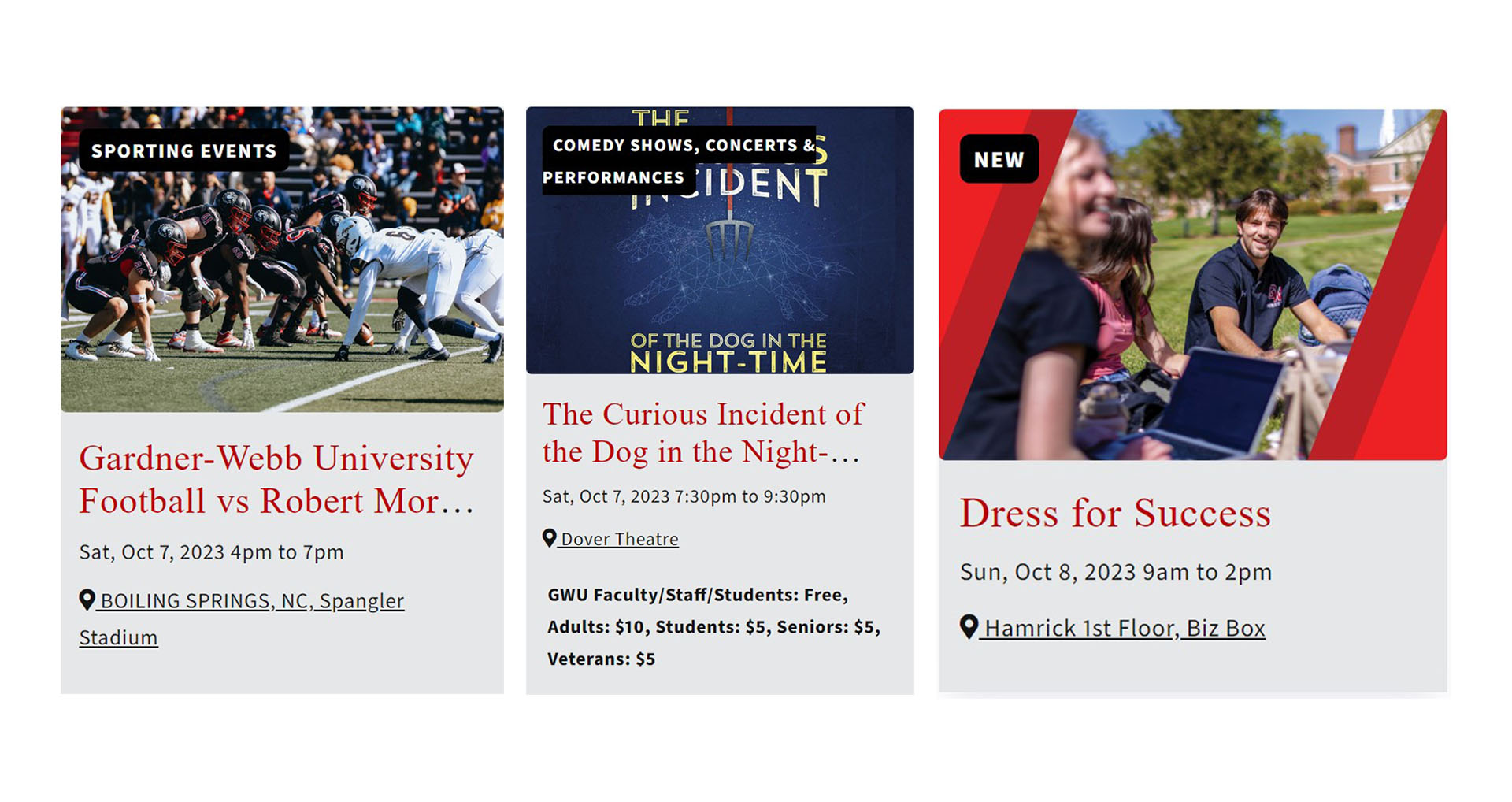**Detailed Caption:**

The image is a screenshot of a laptop screen, depicting three distinct event advertisements side by side, separated by white vertical spacers. 

- **Left Section (Sporting Events)**: The top-left portion showcases a photo of football players in a squatting position. The text above the photo reads, "Gardner-Webb University Football vs. Robert Morris." The event is scheduled for Saturday, October 7th, 2023, from 4 p.m. to 7 p.m. The location is specified as Spangler Stadium in Boiling Springs, North Carolina.

- **Center Section (Comedy Shows, Concerts, and Performances)**: The central section promotes "The Curious Incident of the Dog in the Night-Time," listing it as a performance scheduled for Saturday, October 7th, 2023, from 7:30 p.m. to 9:30 p.m. at Dover Theater. The pricing details indicate that the event is free for GW faculty, staff, and students, while the tickets for adults are $10, and students, seniors, and veterans are $5 each.

- **Right Section (Dress for Success)**: The rightmost section features an image of individuals sitting in a plaza or a green area in front of a university building, with a new indication button that reads "Dress for Success." The event is scheduled for Sunday, October 8th, 2023, from 9 a.m. to 2 p.m. at Hamrick First Floor Biz Box (Hamrick spelled as H-A-M-R-I-C-K).

All images are in color with the text in red and smaller subtext in black against a light gray background.